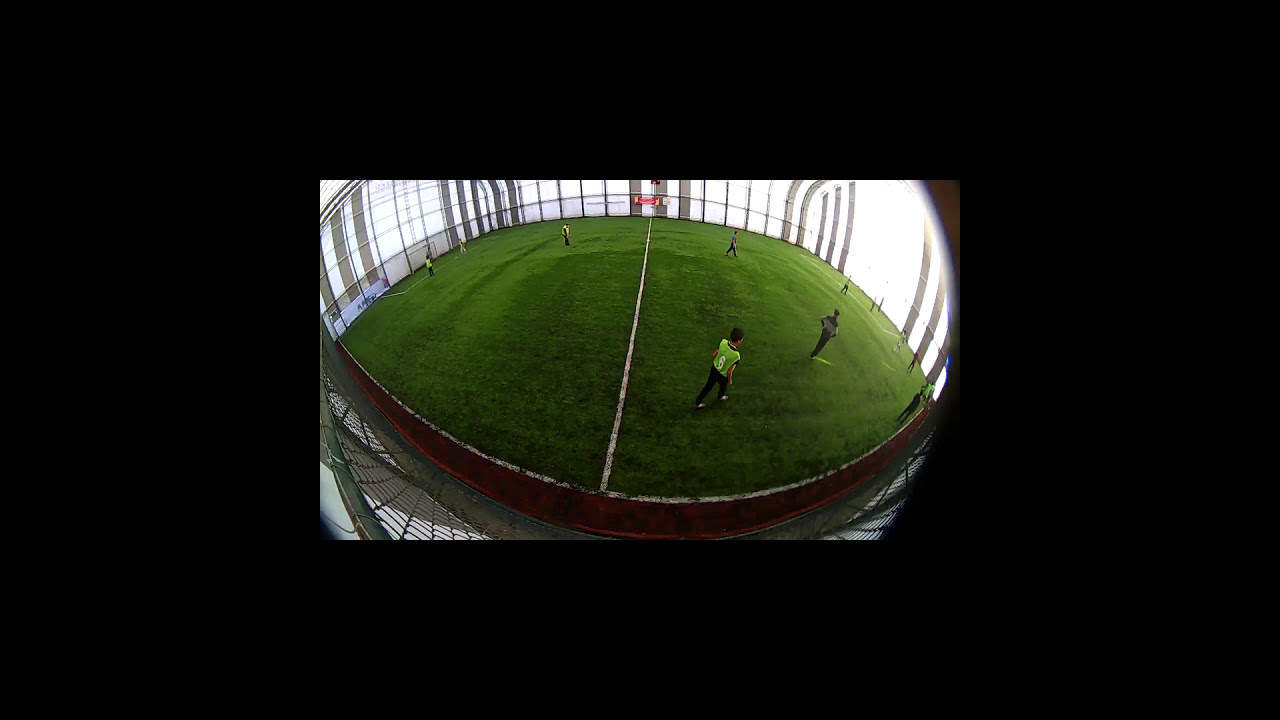The image features a high-contrast composition with a solid black boundary, drawing attention to the central photo, which seems to be a security camera shot capturing an indoor sports field. The vivid green astroturf appears almost artificial against the stark background. Around seven to eight male athletes are scattered across the field, divided into two groups by their shirts—half in neon green and the others in dark or white shirts. The field, enclosed by metal fencing that lets in white light, suggesting an indoor setting, is distorted, possibly due to an ultra-wide or 360-degree lens. This small practice arena is marked with a white halfway line. Despite the indoor setting, the light suggests it might be daytime outside, though the exact conditions are unclear. The players appear to be casually practicing, prepping perhaps for an upcoming game.